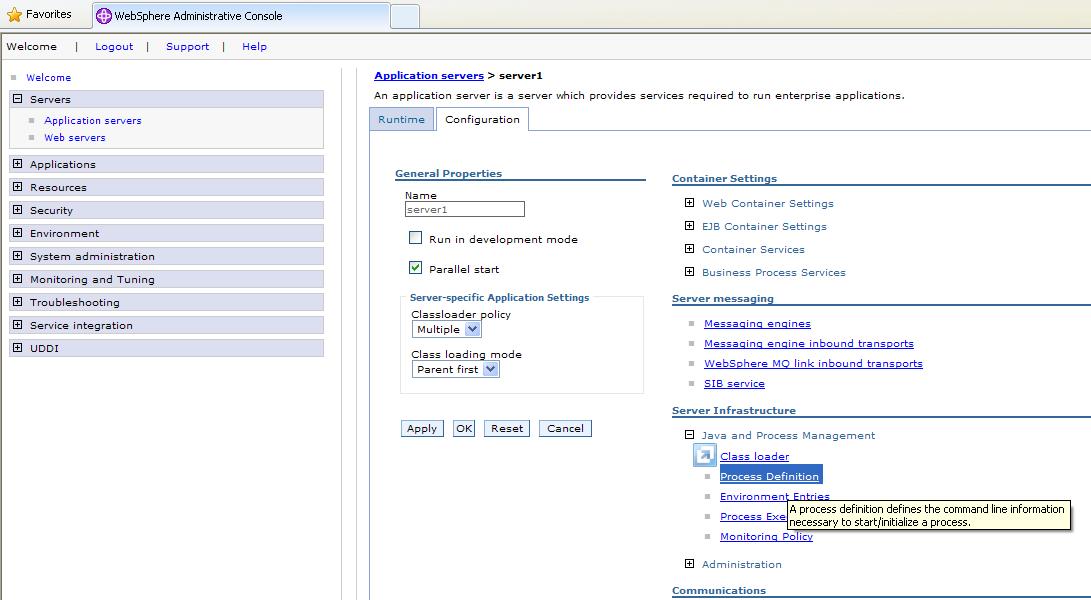The image displays a detailed screenshot of a browser window showcasing the interface of the "WebShare Administrative Console." At the top left corner, two tabs are visible: a "Favorites" tab adorned with a gold star icon, and a "WebShare Administrative Console" tab in black font. Adjacent to these tabs is a small pink-purple circle featuring an unidentifiable white symbol, probably the logo of the application.

Immediately below, a set of four navigation options is displayed: "Welcome" in black, and "Logout," "Support," and "Help" in blue font, indicating that the user is currently on the Welcome page. The page is divided into two primary sections.

On the left-hand side, a pane lists an extensive menu structure. It starts with "Welcome" followed by "Servers," which branches into "Application Servers" and "Web Servers." Below "Servers" are categories such as "Applications," "Resources," "Security," "Environmental," "System Administration," "Monitoring and Tuning," "Troubleshooting," "Server Integration," and "UDDI," each accompanied by a plus icon signifying that additional options can be expanded.

The right-hand side of the screen, occupying roughly 65% of the total area, focuses on details related to "Application Servers." At the top, the navigation path reads "Application Servers > Server1," with "Application Servers" highlighted in blue. Below this path, a brief descriptive sentence explains this section. Two tabs are present under this description: "Runtime," which is highlighted in light blue, and "Configuration," which is white.

Further down, various sections under the "Configuration" tab are displayed, including "General Properties," "Container Settings," "Server Messaging," and "Server Infrastructure," each pertaining to different aspects of server configuration.